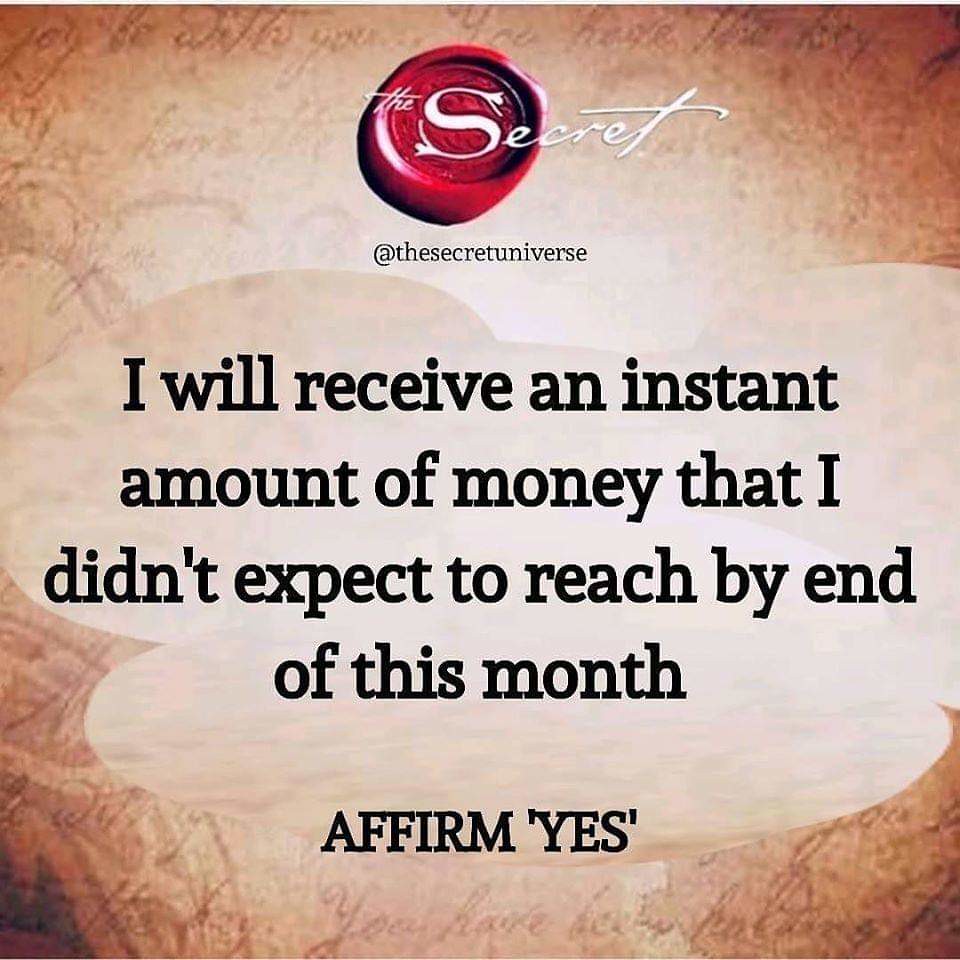This square image prominently displays an inspirational quote as its central focus. The quote, written in bold black text, reads: "I will receive an unexpected amount of money by the end of this month. Affirm." Above the quote, a round red circle bears the words "The Secret" at its top, while below the circle, it says "@The Secret Universe." This design suggests a promise or affirmation connected to the principles outlined in "The Secret," implying that by endorsing this affirmation, one might attract unexpected financial prosperity.